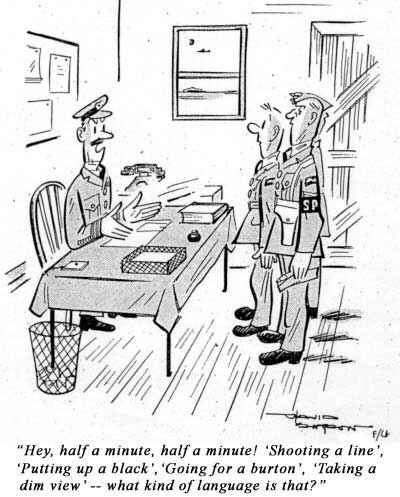The black-and-white cartoon illustrates a scene in a small office with a long table covered by a tablecloth. On the left side of the image, a police officer or possibly a military general, identifiable by his round-brimmed cap and mustache, is seated at the table, which holds various items such as a book, a paper tray, and a few other objects. Opposite him, on the right side, stand two other uniformed men, one with an "SP" armband and a holster at his side. The officer at the desk addresses the men, who appear confused or inquisitive, with the caption positioned at the bottom of the image: "Hey, half a minute, half a minute, shooting a line, putting up a black, going for a Burton, taking a dim view. What kind of language is that?" The detailed black ink drawing captures a moment of communication clearly lost in translation, emphasized by the bewilderment on the standing men's faces.